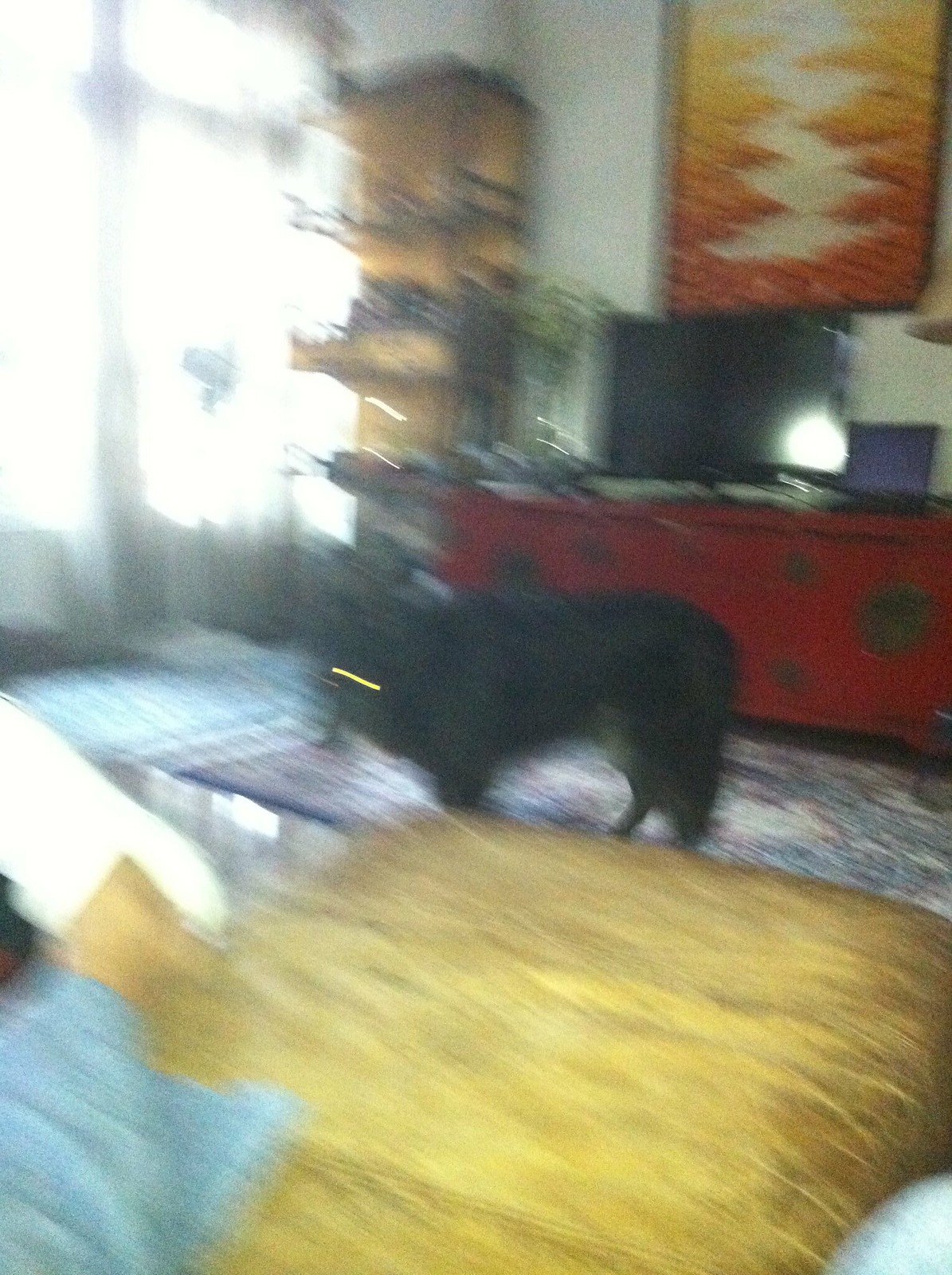In this blurry image, the setting appears to be the living room of a house. A cabinet, located centrally, supports either a TV screen or computer monitor. To the left of this cabinet, there is a shelf, and on the wall behind, you can glimpse a framed picture or painting. The room is bathed in daylight, evidenced by sunlight streaming through partially drawn curtains. In the foreground, a black dog stands attentively in front of the monitor, while a rug lies beneath its paws. The bottom of the image captures a glimpse of a yellow blanket spread out on the floor. The overall scene suggests a cozy domestic atmosphere filled with soft daylight and homely touches.